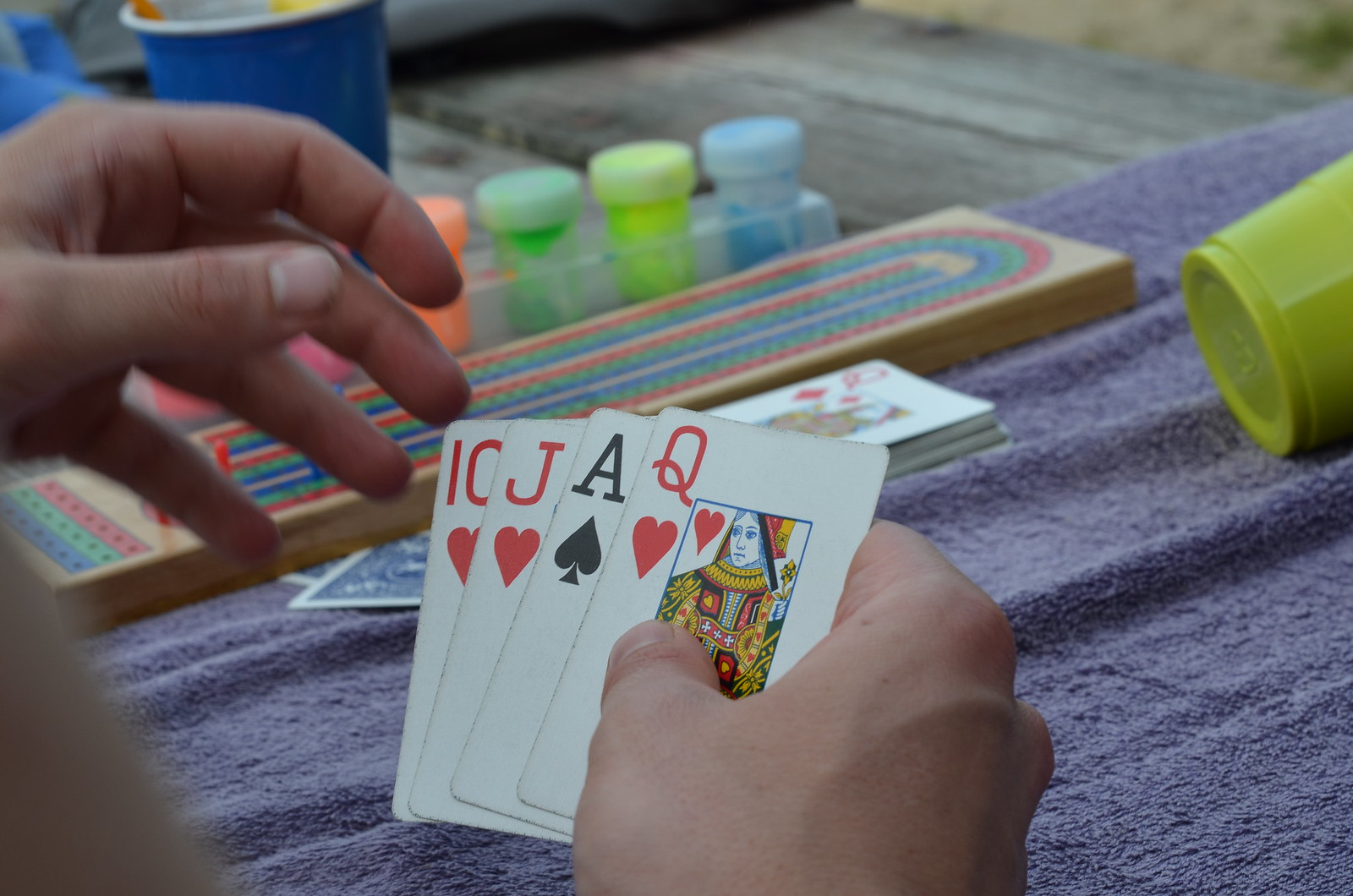In the image, two hands are visible. The hand on the left is held up with fingers splayed, while the hand at the bottom is holding four playing cards. The cards being held are a ten of hearts, a jack of hearts, an ace of spades, and a queen of hearts. Beneath the hands, a bluish-purplish towel is spread out. To the left of the hand displaying the cards, there is a stack of cards with a queen of diamonds on top. On the right, a couple of face-down cards are also visible. The background is highlighted by fluorescent paints, adding vibrant splashes of color to the scene.